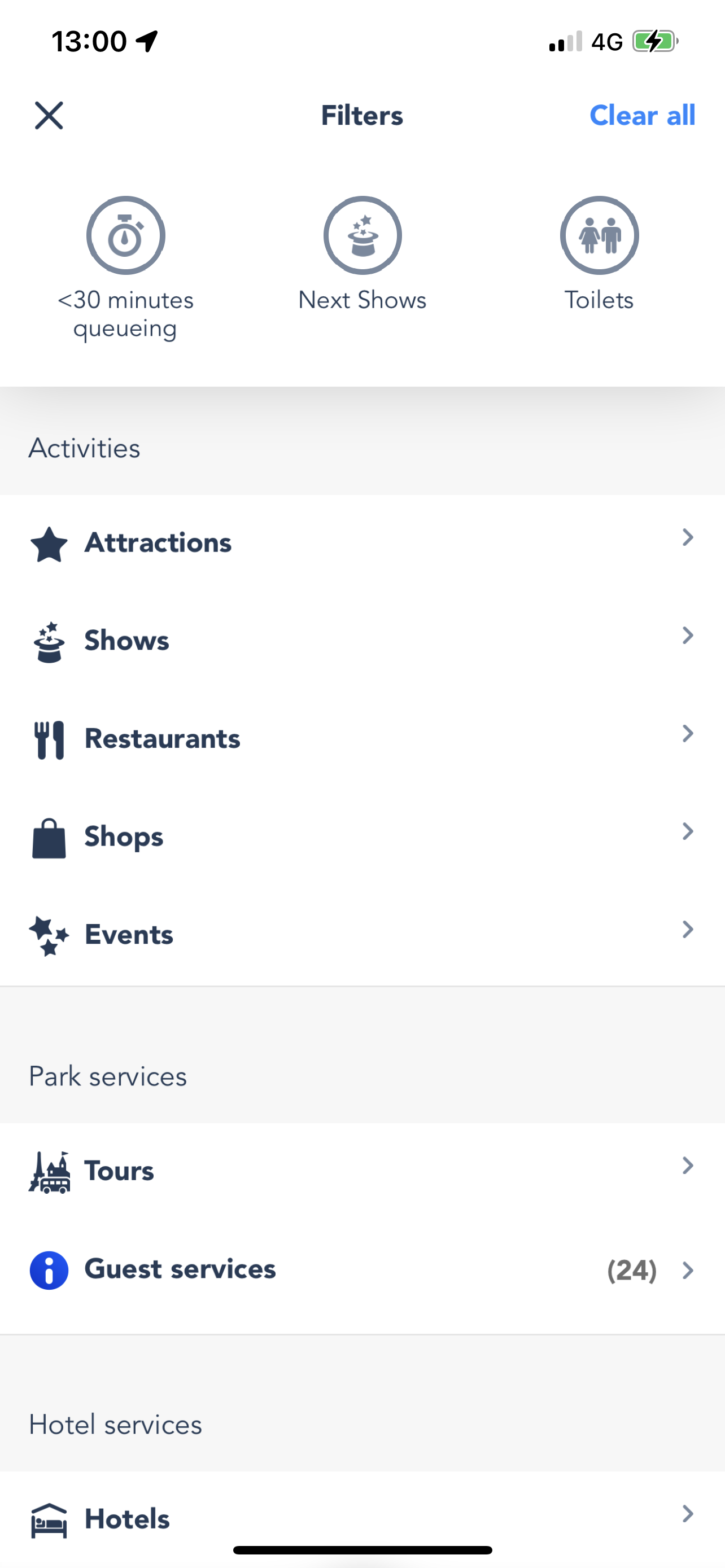The image displays a user interface, presumably of a mobile app or digital screen, with multiple icons and features arranged in a structured layout. 

At the top left, a grey arrow points rightwards next to the number "1300". Adjacent to it is a Wi-Fi signal indicator showing about half strength, accompanied by the "4G" label. Additionally, there is a green battery icon with a black lightning bolt, signaling that the device is charging.

On the next line down, on the left side, there are options labeled "X," "Filter," and "Clear All" in blue font. Below this, a circle encloses a stopwatch icon, with text indicating "greater than 30 minutes queuing" written in black font. 

To the right, another circle features an upside-down magician's hat with a star above it, labeled "next shows." Parallel to this, a grey circle depicts two people, with "toilets" written underneath.

Further details include a light grey box sectioned with various activity options:
- "Activities" on the left
- A black star labeled "attractions" followed by a right-facing arrow
- The magician's hat icon for "shows" followed by another right-arrow
- Fork and knife icon indicating "restaurants" with a right arrow
- Shopping bag icon for "shops" followed by another right arrow
- Three stars labeled "events" followed by another right arrow

Beneath this, another grey box is labeled "park services." Below that, on a white background, there's an image of the Eiffel Tower and a train or bus icon, with the text "tours" followed by a right arrow.

A blue circle with a white "i" symbol indicates "guest services" in black font, followed by "24" in brackets and another right-arrow.

A grey background box, labeled "hotel services" in light grey lettering, depicts an icon of a roof and a bed with a person laying in it, labeled "hotels" in black font. This section is bordered by a black line to the center and a right arrow to the right.